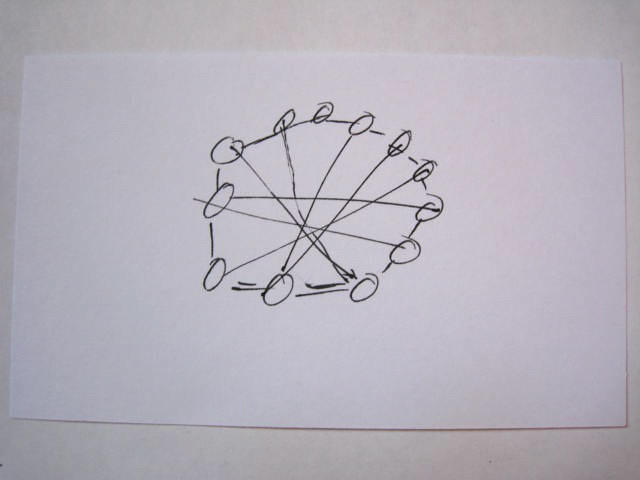In the image, a white piece of paper lies on a light grayish background, casting a shadow primarily along the bottom edge and slightly to the right side. Centrally positioned on the paper is a hand-drawn illustration. This drawing includes several circles arranged to form a larger circular shape. Connecting these circles are a series of lines, some straight and others curved, resulting in a criss-cross pattern that appears somewhat haphazard and irregular. Notably, the lines are more prominent and thicker at the bottom of the drawing, which adds a sense of depth and contrast. The gray background of the image features subtle tonal variations, being slightly darker on the left side, transitioning to a lighter shade in the middle, and then again becoming a bit darker towards the right, although not as dark as the left side.